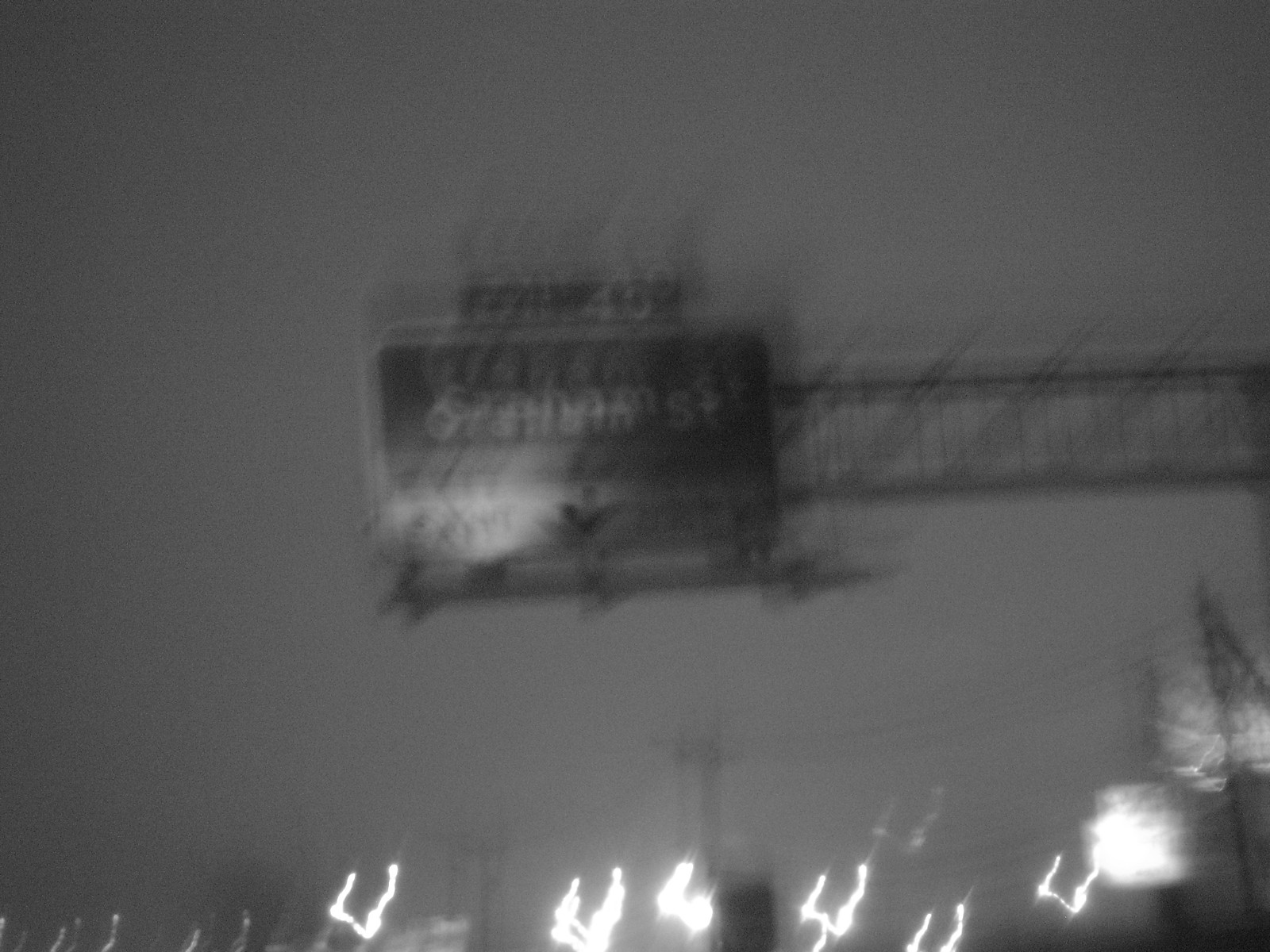In this blurry and grainy evening photograph, the motion blur creates an ethereal effect as lights stretch and pull across the frame. The sky and background are enveloped in a muted grey, characteristic of twilight. Amid the abstracted forms, you can discern outlines of telephone poles and silhouettes of trees, all partially obscured by the sweeping light trails. Illuminated by scattered lights, an overhead street sign on a large arm is faintly visible. Though the green sign is lit, only the text "Exit 40" can be clearly identified, while the rest remains illegible. The image's movement captures a fleeting moment of transition, shrouded in the mystique of dusk.